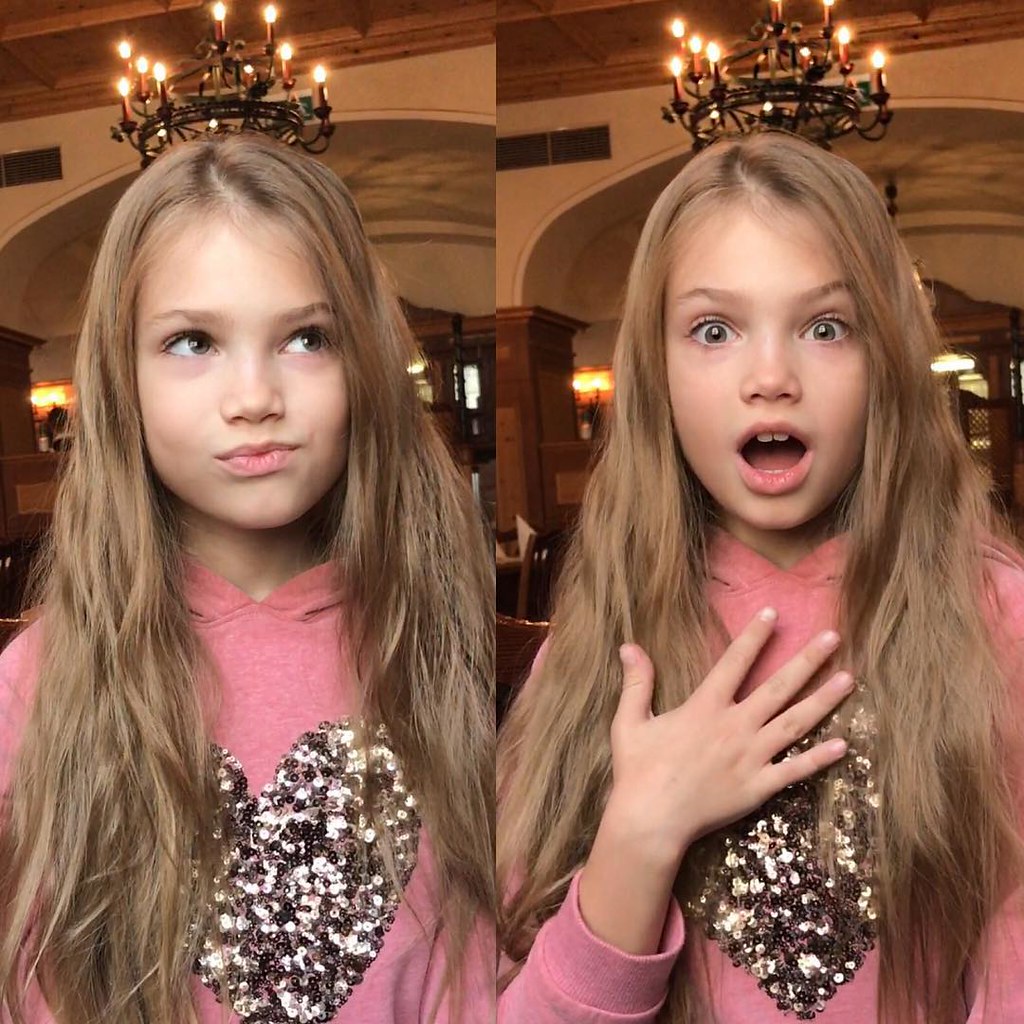This image features a young girl with long dirty blonde hair, captured in two distinct poses. In both, she is dressed in a long-sleeve pink shirt adorned with a sparkly, sequin heart at the center. On the left side of the photo, she gazes up and to the left with her lips slightly pursed, exuding an inquisitive expression. On the right, she displays a shocked expression, her eyes wide and her mouth agape, with one hand placed on her chest. The scene is set in a beautifully ornate room, likely a high-end restaurant or hotel. Overhead, chandeliers illuminate the space, and an elegant white archway extends from a wooden pillar in the background. The high ceiling suggests a spacious and upscale environment, with some light filtering in from further back.